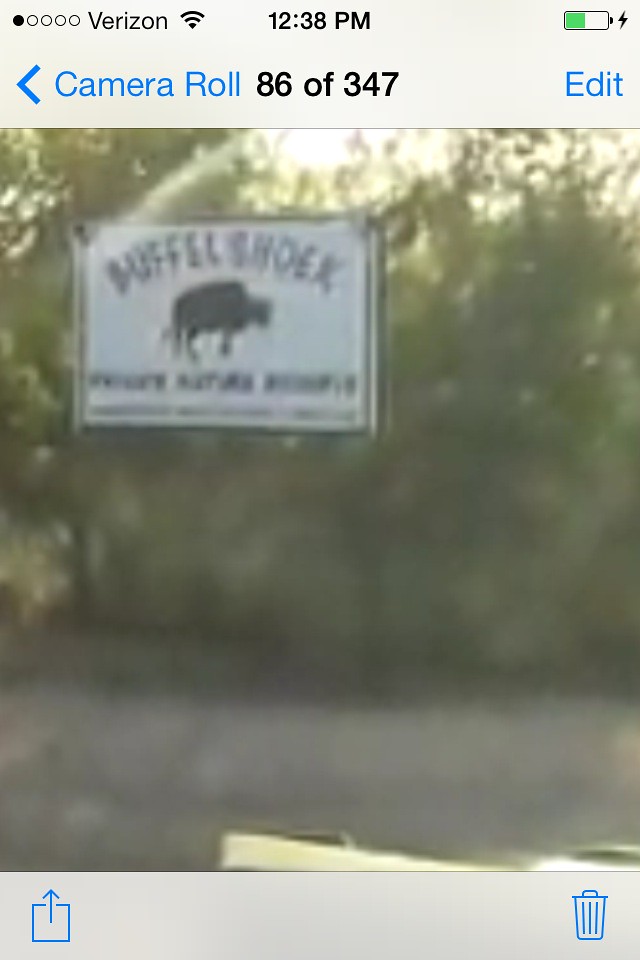Image Description:
A digitally captured image showcasing multiple layers of screens, contributing to its blurry and distorted nature. The photograph displays a signboard, which is difficult to discern due to its poor quality. The image is rectangular, with its longer sides aligned horizontally.

At the very top of the image, there is a grey banner featuring multiple lines of text, though the content is not clearly visible. In the top left corner of the grey banner, there are five circles: one completely black and the remaining are black outlined circles arranged in a row. Next to this, the word "Verizon" is printed in black text, accompanied by an upside-down triangle symbol positioned to its right.

Centrally located on the grey banner, the image shows the time as "12:38 PM" in a clear, black font. Moving to the top right corner, there is an illustration of a battery, depicted sideways. This battery icon is half-filled with green, indicating the charge level, and has a black lightning bolt symbol beside it on the right.

Beneath the grey banner, blue text reads "Camera Roll," and following that, black text shows "86 of 347," indicating the position and total number of images in the photo gallery.

Overall, the unclear quality combines physical characteristics of a physical screenshot taken from a phone, which itself is an image displayed within a phone gallery.